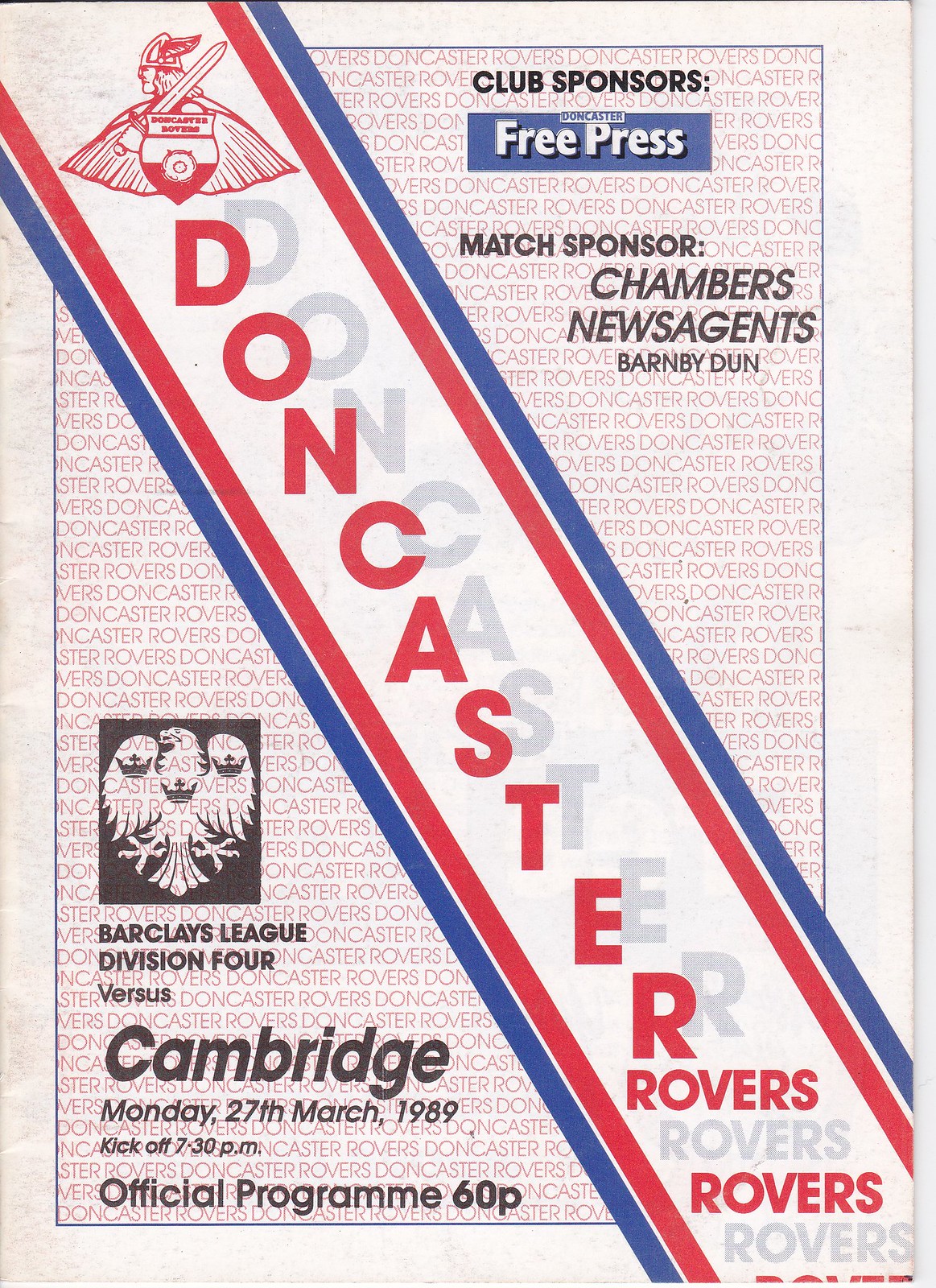The image depicts the front cover of a vintage magazine or program from the 1980s, dedicated to a football match. Dominating the cream-colored background, the cover features a prominent white banner running diagonally from the top left to the bottom right, bordered by blue and red stripes. This banner prominently displays "Doncaster Rovers" in large red letters, with a subtle gray shadow repeating the text behind it. The background is filled with a recurring "Doncaster Rovers" text in light red. 

At the top center, "Club Sponsors" is printed in black, followed by a blue rectangular shape containing "Free Press" in white. Below this, "Match Sponsor Chambers News Agents Barnby Dunn" is listed in black. The upper right corner showcases a red shield logo with a Viking, who is side-profiled, wearing a winged helmet and holding a sword.

In the bottom left corner, there is an additional logo of an eagle with outstretched wings, adorned with three small crowns—one on its chest and one on each wing. Adjacent to the eagle, important match details are provided: "Barclays League Division 4 vs. Cambridge, Monday, 27th March 1989, kickoff at 7:30 p.m., official program, 60p," all printed in black. The entire cover is framed with a white edge, contributing to the classic and organized layout of the magazine.